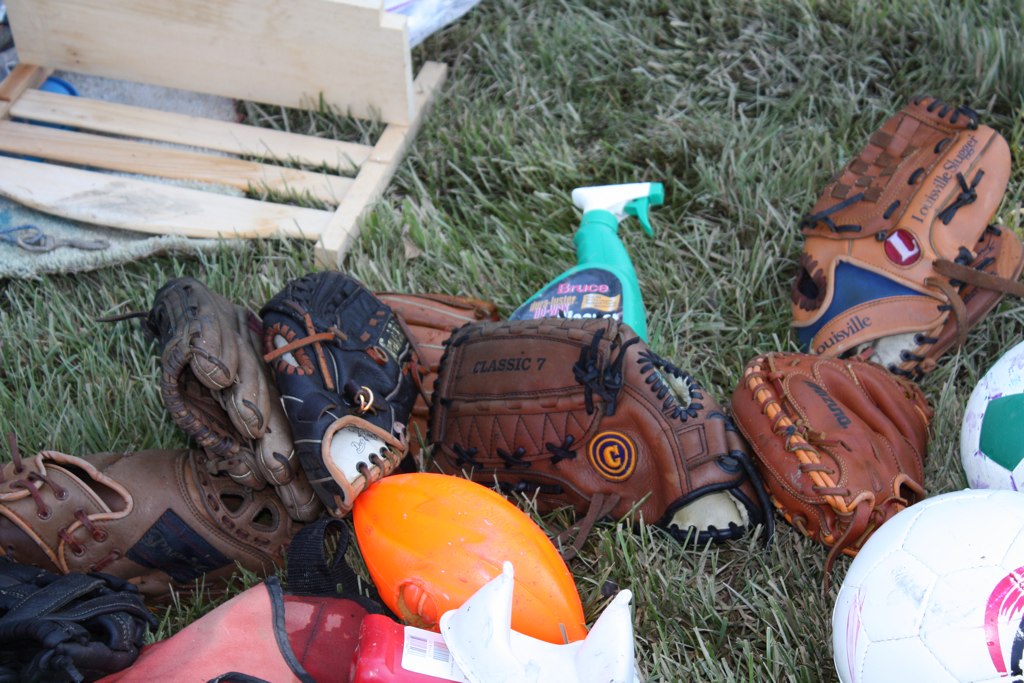The photograph taken outdoors showcases an assortment of sporting equipment scattered on a patch of medium-length grass that is somewhat untended. Dominating the scene are seven baseball gloves in various shades of leather, from black to light brown, highlighting differences in shapes, brands, and sizes. Also visible are two soccer balls: one white with green panels, the other white and purple. An orange Nerf football lies prominently among the items. To the upper left corner of the image, there is an unfinished wooden structure that could be part of a chair or bench, potentially made from pine. A green spray bottle with a white cap is also seen, likely intended for cleaning the gloves. Additionally, there seems to be a red and white object, possibly a bag, in the mix. The wooden structure rests over a piece of plastic, adding to the casual disarray of the scene.